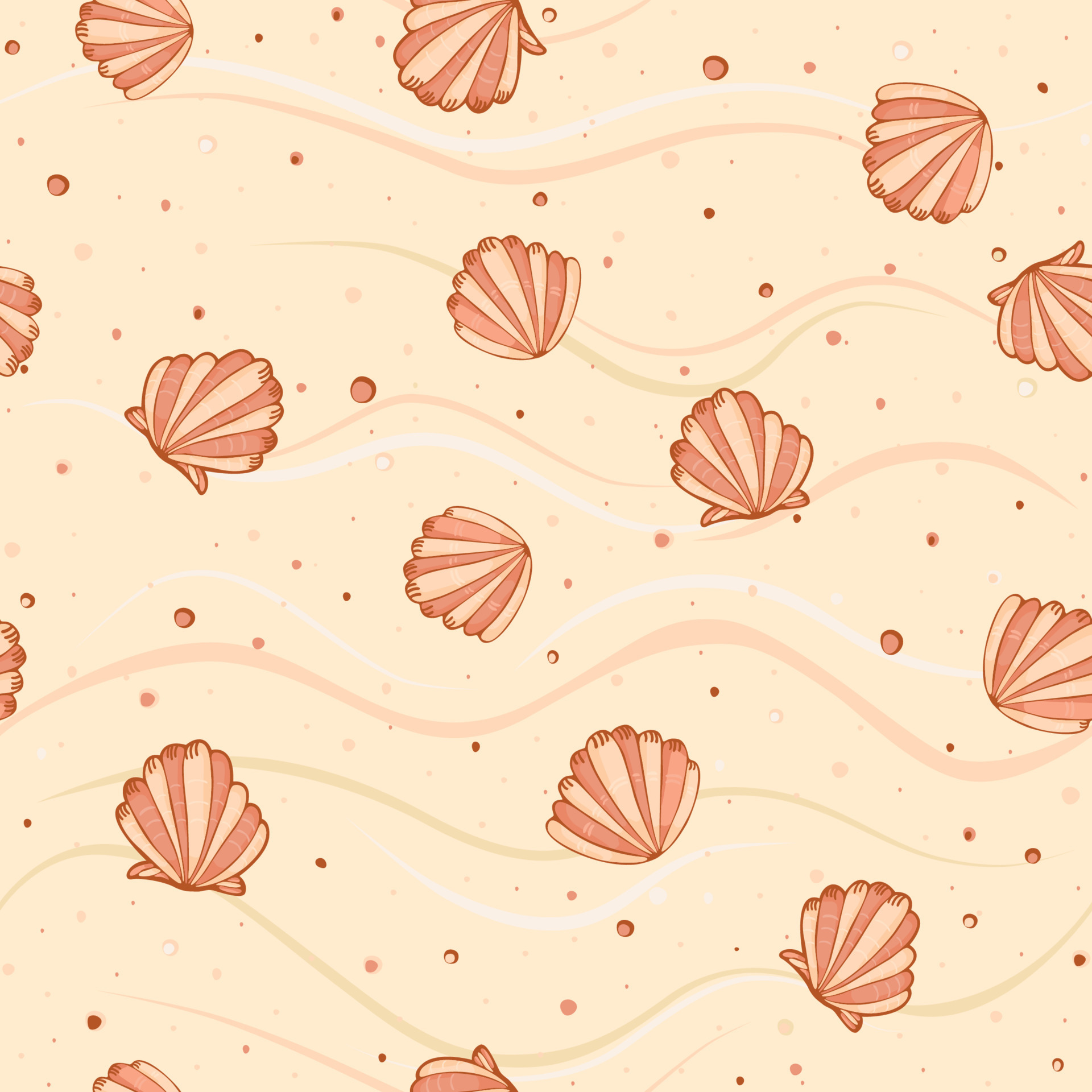The image appears to be a digitally created illustration of wallpaper featuring a repeated pattern of seashells. The background is a tan color with a mix of light green and white squiggly lines, as well as numerous pink dots and circles that simulate bubbles. Dominating the design are seashells in shades of pink, alternating between dark red and light beige stripes, arranged in various directions that create a dynamic and somewhat random pattern. There are approximately 12 to 14 seashells visibly dispersed across the image, with some shown in full and others partially visible, enhancing the impression of a continuous wallpaper design. The overall effect is abstract and impressionist, evoking a sense of underwater scenery with its scattered bubbles and wavy lines.